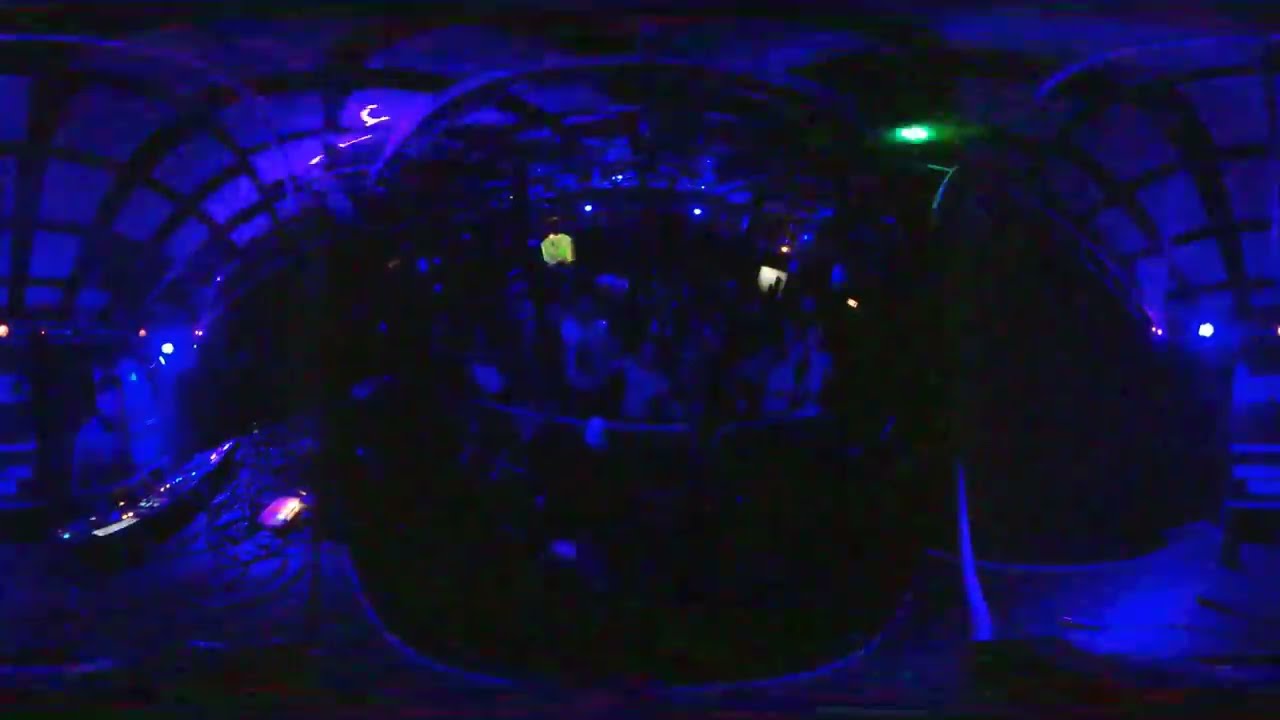In this dark and distorted image, predominantly colored in deep blues and blacks with intermittent green light, we see a nightclub scene. Centered in the image, behind a round post barrier, a group of people wearing mostly white shirts appear to be congregating, likely enjoying the performance. To the left side of the image, a DJ stands behind a turntable or soundboard setup, with equipment buttons illuminated. Fluorescent green lighting sharply points towards the center from the left, indicating special lighting, possibly a strobe. The image is crisscrossed by curved lines resembling ceiling beams that arc towards the center from both sides. In the top right corner, white letters "N" and "V" are visible, along with a tiny white speck near the right border, adding a subtle detail to the scene.